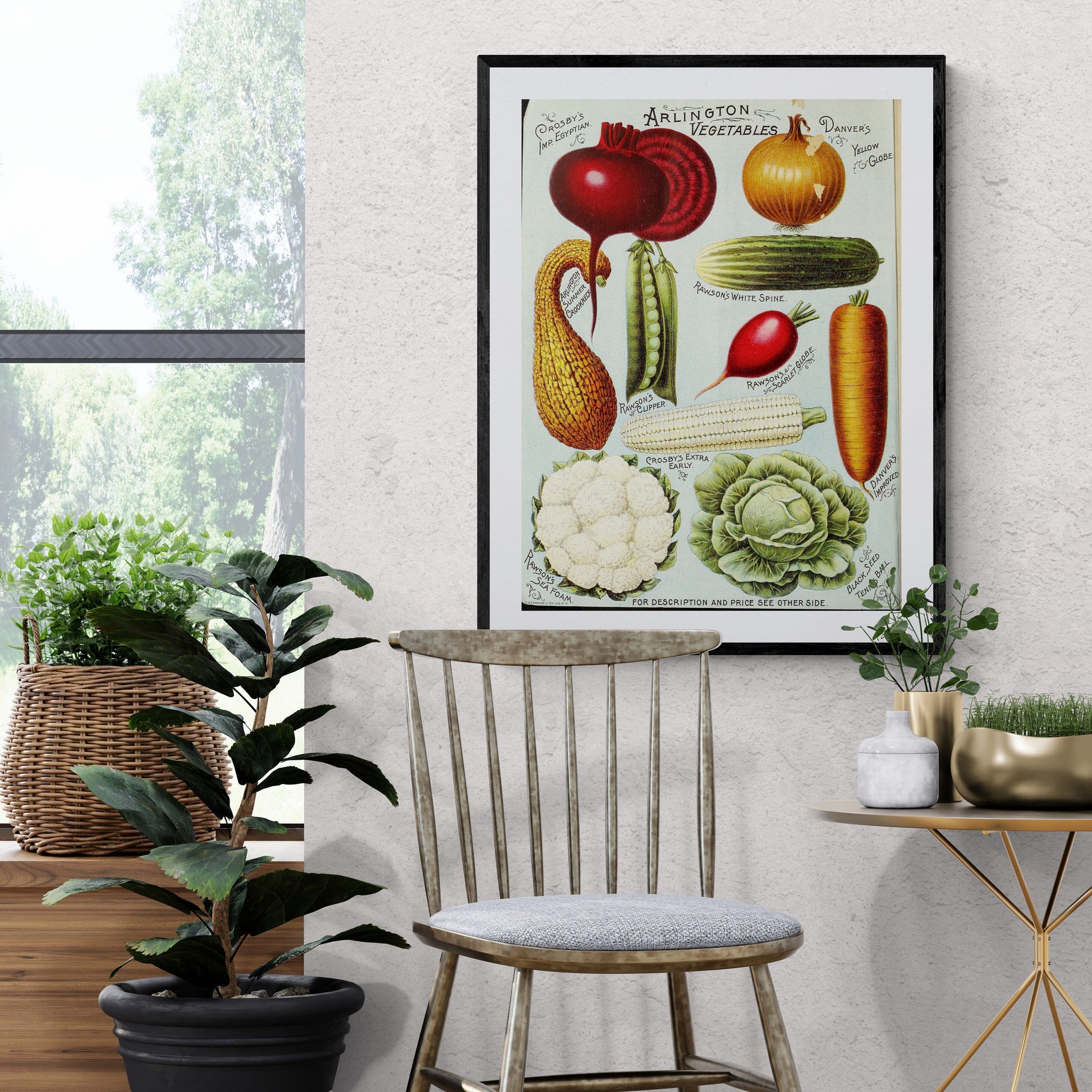The photograph captures a rustic kitchen scene with a cozy and eclectic layout. On the left, a third of the image is dominated by a window, through which nature is visible. Beneath the window is a brown box or shelf that supports a rattan basket housing a green plant. In front of this, a rubber tree in a dark charcoal gray pot sits at the corner of a white wall. Adjacent to the rubber tree is an old-fashioned gray wooden chair with a light gray cushion.

Behind the chair, affixed to the textured white wall, is a vibrant painting labeled "Arlington Vegetables." This artwork is richly detailed and features an assortment of vegetables such as carrots, onions, cucumbers, cauliflower, lettuce, corn, and beets, depicted in an array of colors from red and green to yellow and orange.

To the right of the chair and in the bottom-right corner of the photograph is a small, elegant table with legs that converge at the middle and spread outward at the floor. This table holds two silver pots; one filled with eucalyptus leaves and the other is a low bowl pot housing small grass and a covered pot. The scene blends traditional and contemporary elements, creating a warm and visually engaging atmosphere.